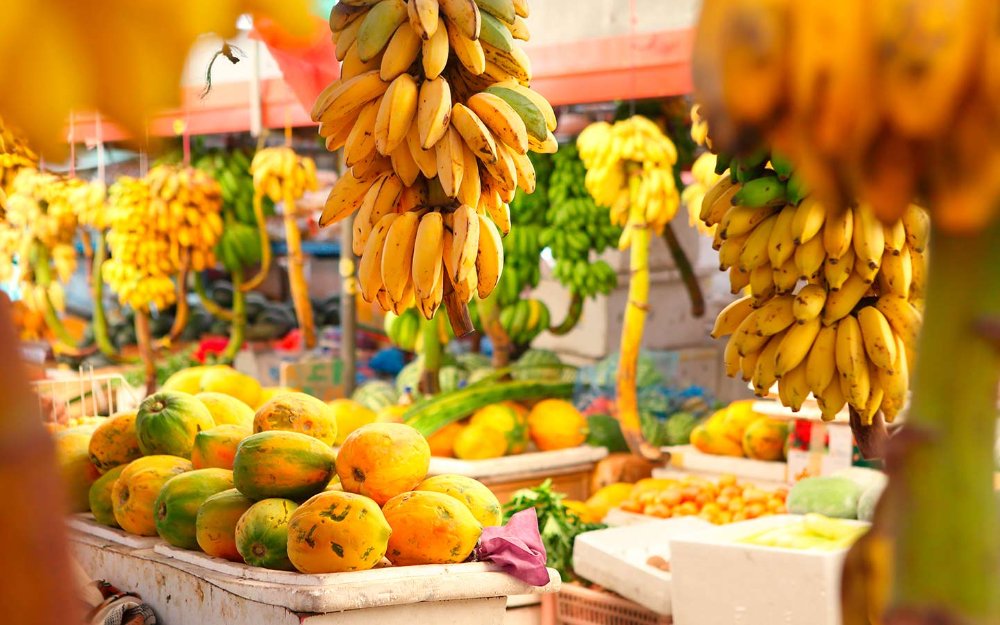This vibrant photograph captures a bustling tropical fruit market brimming with a variety of colorful produce. In the foreground, numerous bunches of bananas, predominantly yellow with some green, hang from structures supporting an orange awning above. Some bananas appear out of focus, adding depth to the scene. Below the hanging bananas, white baskets brim with yellow and green mangoes and other assorted fruits, including orbs of oranges and melons in shades of yellow, green, and orange. Scattered boxes and crates further contribute to the organized chaos of the market. The background reveals more stacks of green and yellow bananas, hinting at the market's vast inventory. The scene is characterized by colorful awnings supported by vertical poles, and even a rustic pink structure in the distance. Elements of purple, likely from napkins or tissue paper, subtly complement the yellow and green hues of the mangoes, adding an extra pop of color to this richly detailed, bountiful display. No individuals are present, suggesting a moment captured either before the market opens or during a quiet period, with all the fruit meticulously arranged and ready for sale.